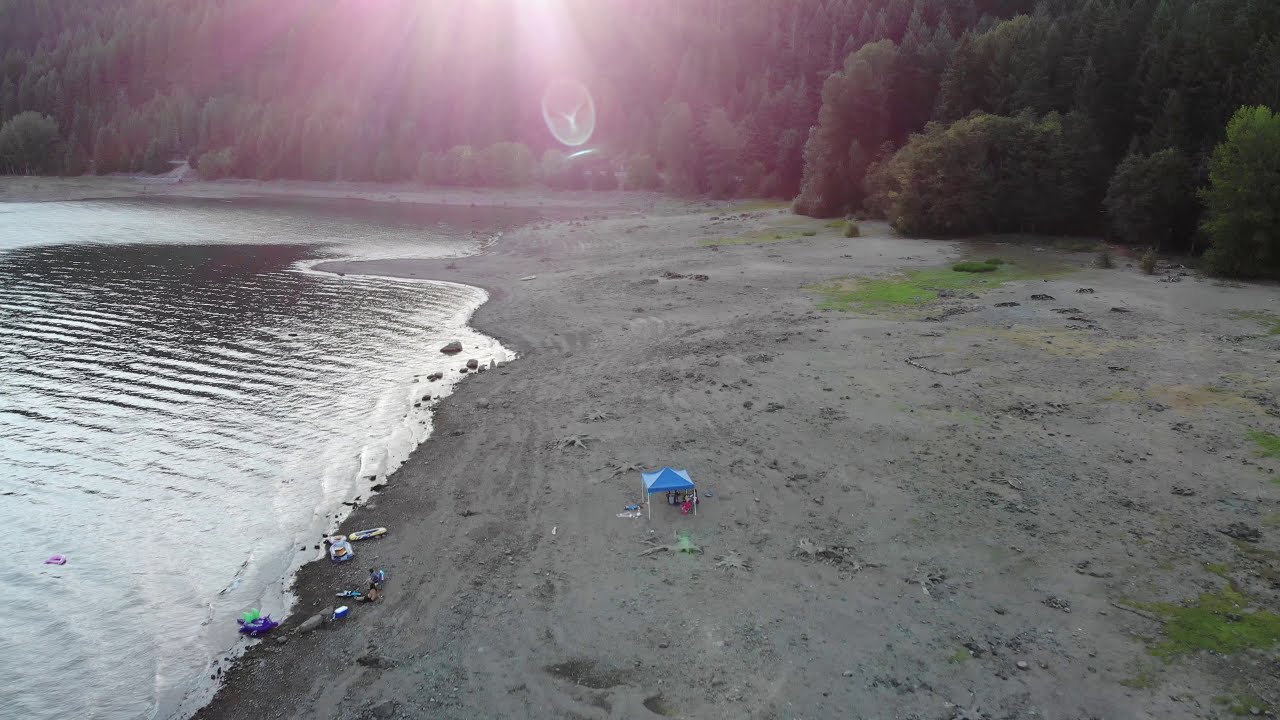A photograph taken from a high vantage point, perhaps a cliff, captures a serene shoreline that appears to be part of a lake or river. The image, likely taken either early in the morning or late in the afternoon due to the limited light, features a gray sandy beach that weaves through the landscape. On the left, the body of water ripples gently, while the right side is bordered by a dense forest of tall trees stretching from the top left to the right. Near the bottom of the image, the shore is populated by small figures who seem to be engaging with water equipment, possibly surfboards, canoes, or inflatable boats. Central to the scene is a blue-tinted canopy, suggesting a small gathering under its tent-like structure. The sandy beach extends back into the scene, merging with the natural beauty of the surrounding area. The overall ambiance is tranquil, marked by a soft lens flare from the setting or rising sun, casting gentle rays across the photograph.